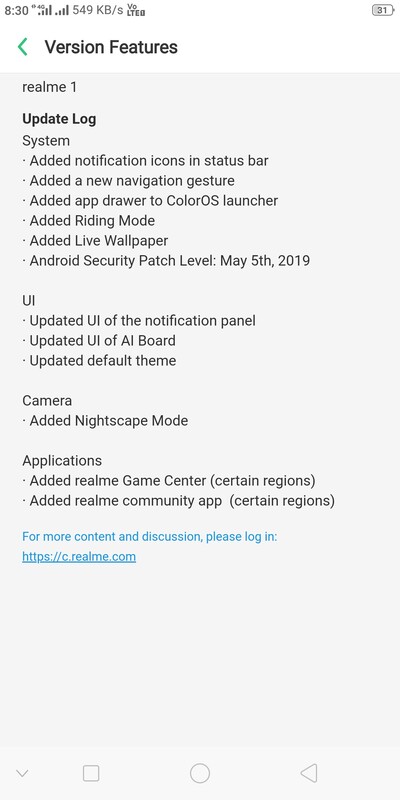This image is a screenshot of a smartphone displaying the "Version Features" tab under the settings screen. At the top of the screen, the time reads 8:30, and the phone shows full service with all signal bars completely filled. The screen highlights various updates and features categorized systematically in an update log titled "Realme 1."

The first main category is "System," which lists:
- Added notification icons in the status bar
- Added a new navigation gesture
- Added an app drawer to the ColorOS launcher
- Added a writing mode
- Added live wallpaper
- Android security patch level updated to May 5th, 2019

The next main category is "UI," detailing:
- Updated UI in the notification panel
- Updated UI of the AI board
- Updated the default theme

Following the UI improvements is the "Camera" section, which notes:
- Added Nightscape mode

Lastly, the "Applications" section includes:
- Added Realme Game Center (available in certain regions)
- Added Realme Community app (available in certain regions)

At the bottom of the screen, there is a prompt in blue text encouraging users to visit "www.c.realme.com" for more content and discussion.